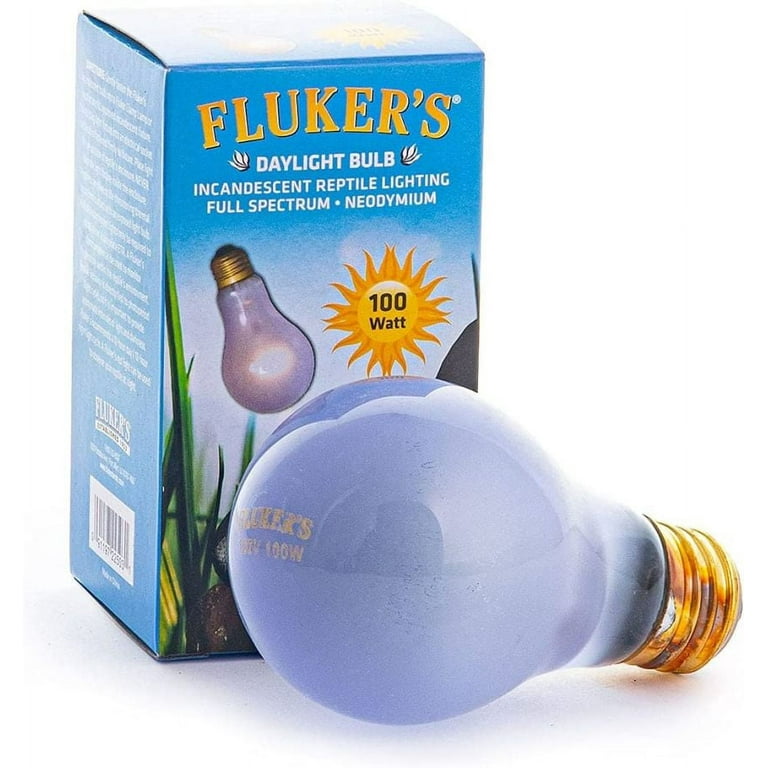The image is a detailed advertisement for a "Flocker's Daylight Bulb," designed specifically for reptiles. Central to the image is the full spectrum neodymium 100-watt incandescent bulb, showcasing its bluish glass that mimics daylight wavelengths. The bulb features a brass-colored screw base and is prominently displayed in front of its original packaging—a rectangular box approximately twice as tall as it is wide.

The box, made from thin cardboard and predominantly blue in color, serves as a backdrop that emphasizes natural elements like greenery and a subtle lizard image, enhancing the product's appeal to reptile owners. The glass portion of the bulb is positioned towards the viewer, highlighting a central sun graphic with "100-watt" printed in bold black letters. The packaging also features an image of the bulb, oriented downward, mirroring the real bulb's position.

On the left side of the box, visible text presumably details the benefits of the light bulb for reptiles, reinforcing its purpose. At the bottom left corner, a white rectangle contains the barcode. Overall, the photograph captures both the product and packaging meticulously, conveying essential details about the "Flocker's Daylight Bulb" and its benefits for reptile lighting needs.